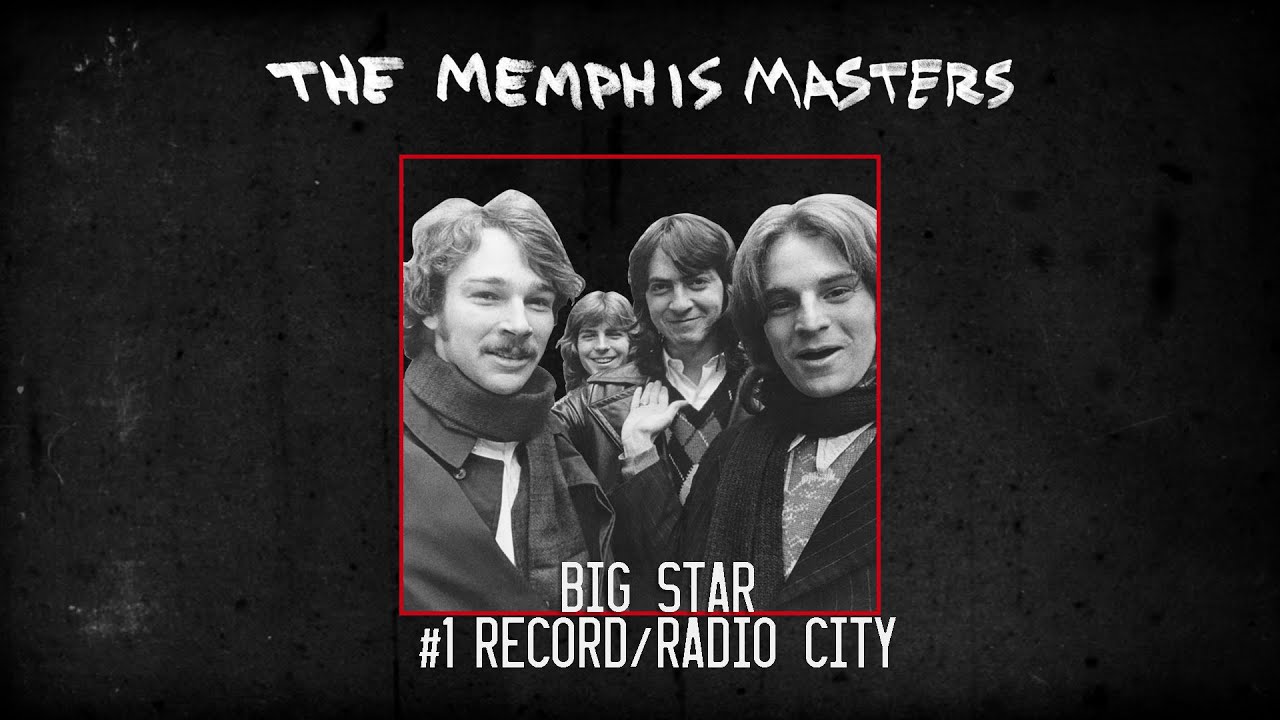The image is a vintage-style advertisement for the band Big Star and their albums *#1 Record* and *Radio City*. The poster features a distressed black wall background that gives it a textured, aged look with scuff marks and scratches. At the top of the poster, in bold white text that appears hand-painted, are the words "The Memphis Masters." Below this text, within a red rectangular outline, is a black and white photograph of the band members. The photo shows four men dressed in typical 1970s attire, including scarves, coats, sweater vests, and collared shirts, all smiling at the camera. Beneath the red-outlined box, in printed white text, it reads "Big Star #1 Record / Radio City." The red square only covers about one-third of the advertisement's width, leaving much of the background exposed. The overall design combines a nostalgic aesthetic with a clear emphasis on the band and their celebrated albums.